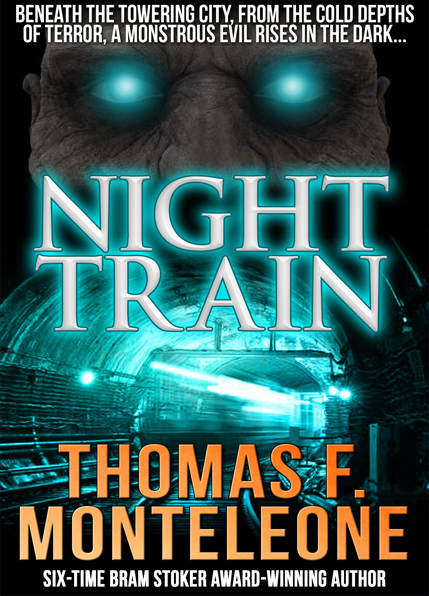The image is the front cover of a rectangular book titled "Night Train." Dominating the cover is a photograph of a round-shaped subway tunnel with a speeding train, blurred by motion and illuminated by an eerie light green hue. Above the tunnel image is a striking depiction of a sinister, zombie-like creature featuring a ghoulish, gray and black face, with only the glowing eyes visible, matching the tunnel's greenish tint. At the top of the cover, in white letters, it reads, "Beneath the towering city, from the cold depths of terror, a monstrous evil rises in the dark." The title "Night Train" is prominently displayed in large white font across the middle of the cover. Beneath the tunnel, in bold orange letters, is the author's name, "Thomas F. Monteleone," followed by a subtitle in white letters that states, "six-time Bram Stoker Award-winning author." The background of the cover is predominantly black, contrasting sharply with the other colors, including shades of light blue, gray, and tan.